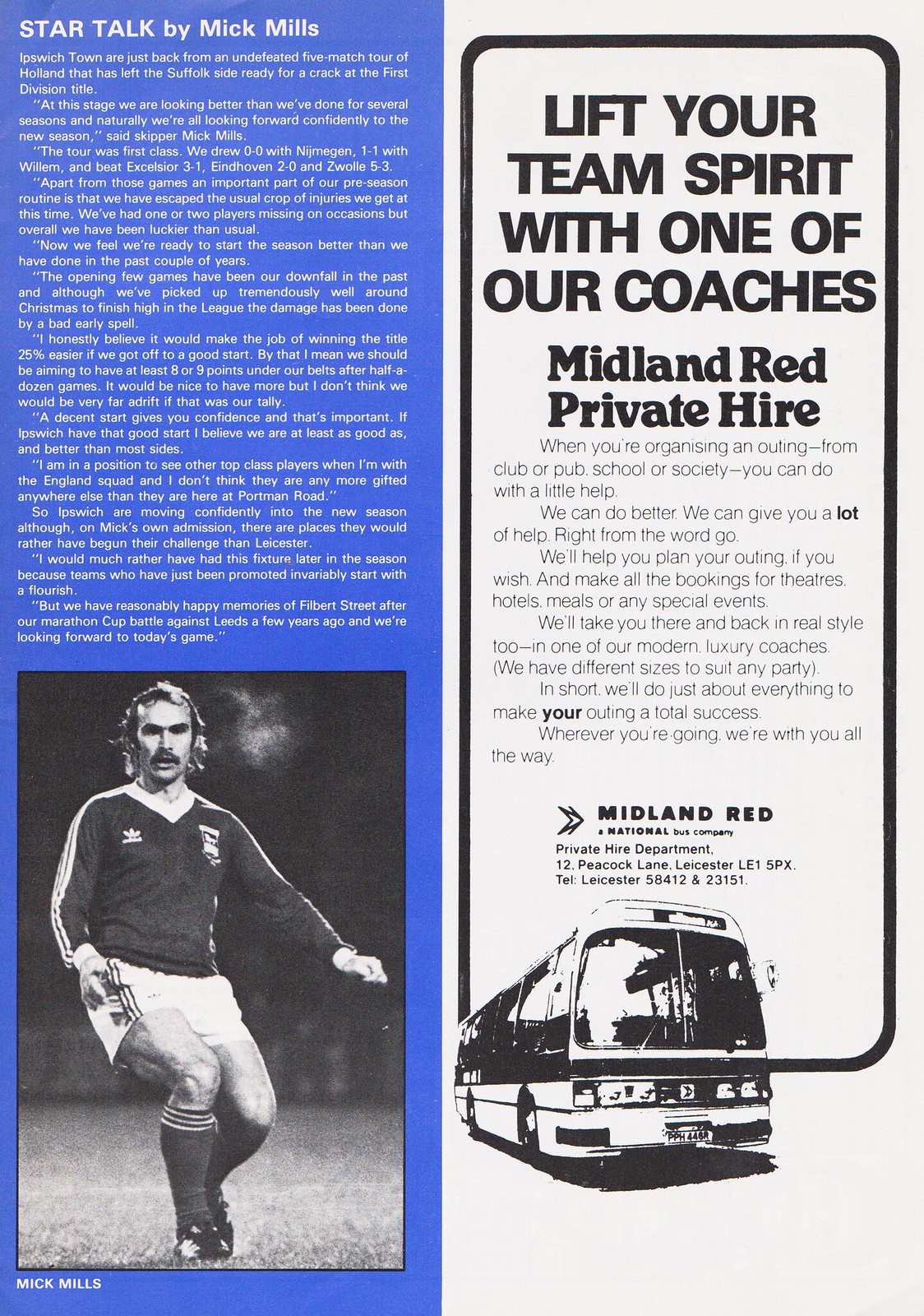The image is a scanned magazine page divided into two vertical columns. The left column has a blue background with the header "StarTalk" in white, uppercase letters, followed by "by Mick Mills" in lowercase. Below this header is a block of white text on the blue background, which is partially unreadable due to small font size. Below the text is a black and white photograph of Mick Mills, a sports player, identified as such at the bottom left corner of the image in white text. Mick Mills is wearing a dark-colored Adidas shirt with two white stripes down the arms, white shorts likely also Adidas, long dark socks with three white stripes, and football boots. He has a moustache and long hair flowing behind him, and he's depicted slightly kneeling forward with both knees bent and arms down in front of him on a grass football pitch, with his breath visible in the nighttime air, indicating it might be cold.

The right column features an advertisement with black text on a white background encased in a black box. Prominently displayed within it is bolded text that reads, "Lift your team spirit with one of our coaches, Midland Red Private Hire." The ad promotes organizing outings for clubs, pubs, schools, or societies, offering comprehensive planning services from booking theatres, hotels, meals, to special events. It emphasizes traveling in modern luxury coaches of various sizes suitable for any party. Contact details are provided at the bottom: National Bus Company, Private Hire Department, 12 Peacock Lane, Leicester, LE1 5PX, with telephone numbers Leicester 58412 and 23151. There is a black and white outline of a coach bus at the bottom, next to the text, "Midland Red" and an arrow pointing to the right.